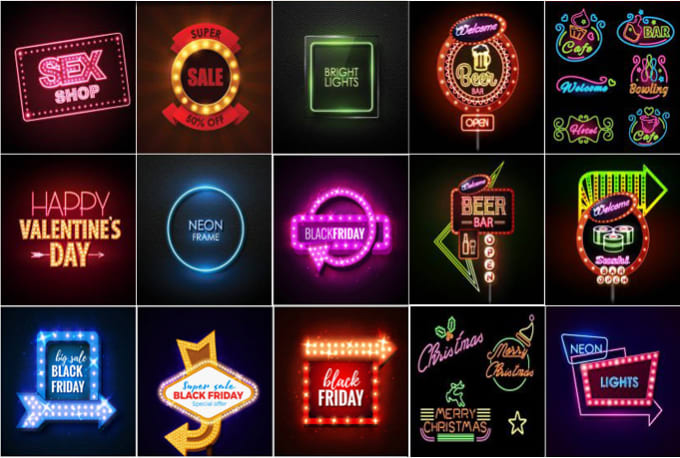The image showcases 15 vibrant neon signs, each displayed within uniform black-background squares arranged in three rows of five. The neon signs, characterized by bright pink, yellow, green, blue, and purple hues, advertise various messages and products. Notable signs include "Sex Shop" with a pink border and text, "Super Sale," "Beer Bar," and multiple signs highlighting "Black Friday" and "Big Sale" in different styles. The signs represent an array of themes such as bars, sales events, and holidays like Happy Valentine's Day. The prominent "Black Friday" sign features an arrow pointing to the right, adding a striking element to the display. The colorful and diverse neon signs suggest an advertisement for a store specializing in customizable neon products.